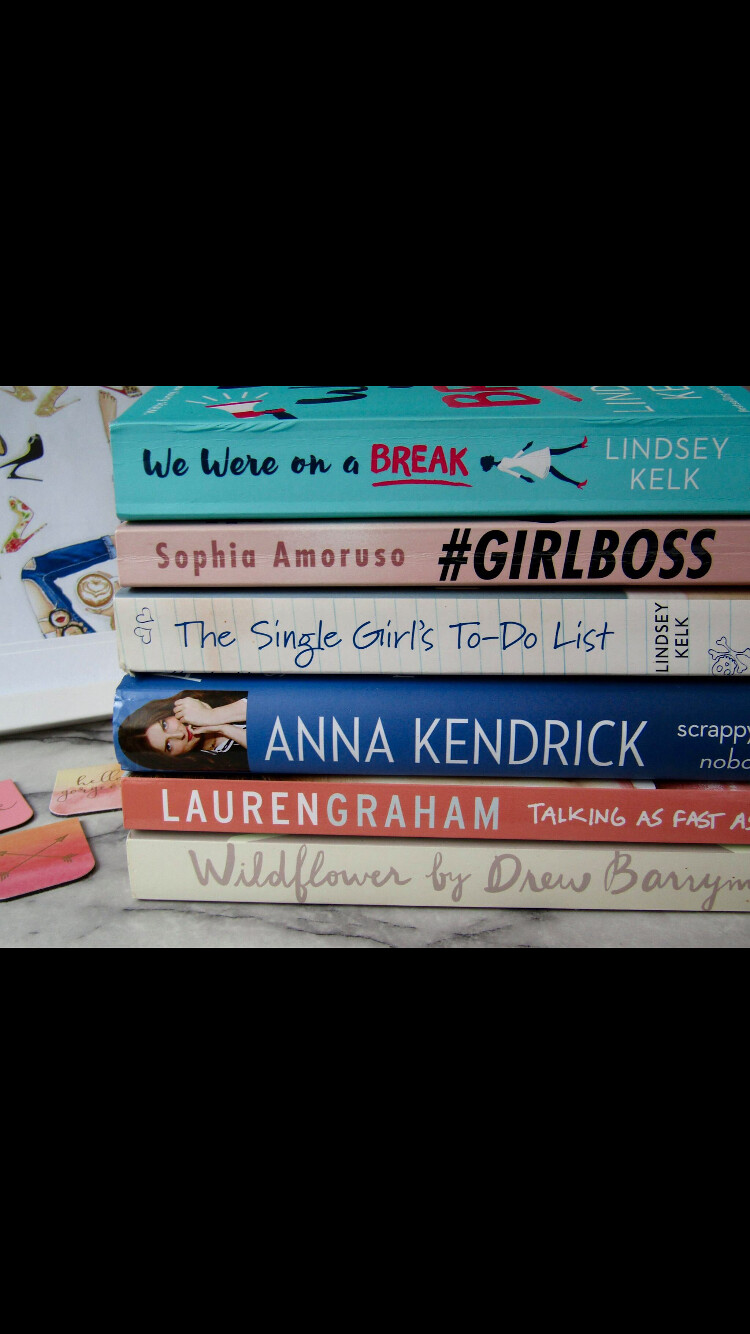The image features a rectangular photograph of a neatly stacked pile of six books placed on a marble surface. The photograph, framed by black headers and footers that each take up about one-third of the image, centers on the books. At the top of the stack, a teal blue book titled "We Were on a Break" by Lindsey Kelk showcases its cover featuring a woman in a white dress and red high-heeled shoes, with "We Were on A" in blue and "Break" in red, underlined. Below it, a pastel pink book by Sophia Amoruso displays the title "#GIRLBOSS" in black print. The third book down is a white cover with blue lettering, titled "The Single Girl's To-Do List" by Lindsey Kelk. Following that, a blue spine with white text reads "Anna Kendrick" and features her image, though the partial title appears to be cut off. The fifth book, characterized by its red spine and white text, is "Talking as Fast as I Can" by Lauren Graham. At the bottom of the stack, "Wildflower" by Drew Barrymore is visible on a light-colored spine. The photograph also includes stickers to the left and illustrated shoes on a card or paper at the top left, further detailing the cozy scene.